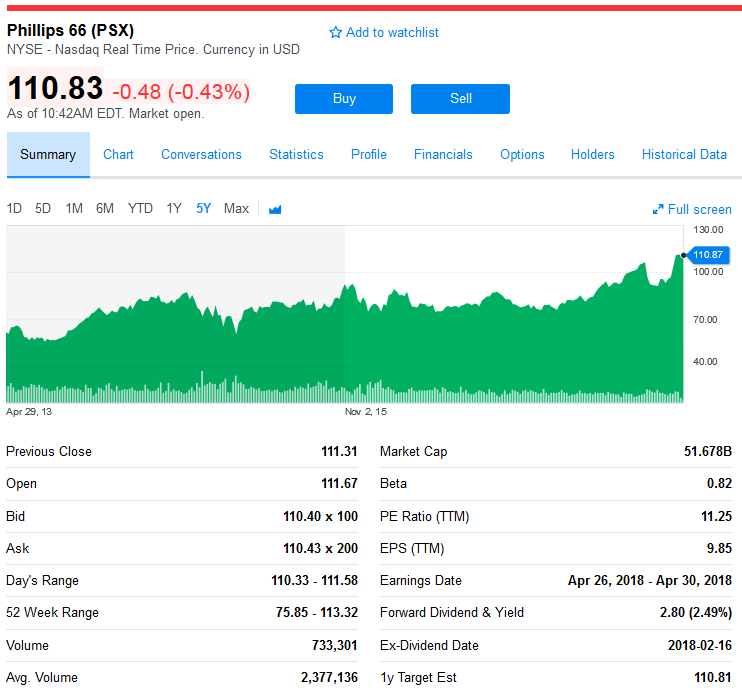The image depicts a stock information page for Phillips 66, trading under the symbol "PSX." The details are displayed with a real-time price in U.S. dollars, as listed on the New York Stock Exchange NASDAQ. At the top center, users are given the option to add this stock to their watch list, highlighted in blue.

The current stock price is \$110.83, reflecting a decrease of \$0.48, or 0.43%, as of 10:42 EDT during market opening hours. Central to the page are blue buttons allowing users to either buy or sell the stock, situated just beneath the 'Add to Watch List' option.

Below these options, a variety of sections are available for in-depth analysis: Summary, Chart, Conversations, Statistics, Profile, Financials, Options, Holders, and Historical Data. Following these sections is a fluctuating green graph illustrating the stock's performance, with data spanning from April 29, 2013, to November 2nd of an unspecified year, ending at a value of \$110.87.

The bottom portion of the image lists comprehensive statistics, including Previous Close, Open, Bid, Ask, Day's Range, 52-Week Range, Volume, Average Volume, Market Cap, Beta, PE Ratio, EPS (Earnings Per Share), Earnings Date, Forward Dividend & Yield, Ex-Dividend Date, and a One-Year Target Estimate.